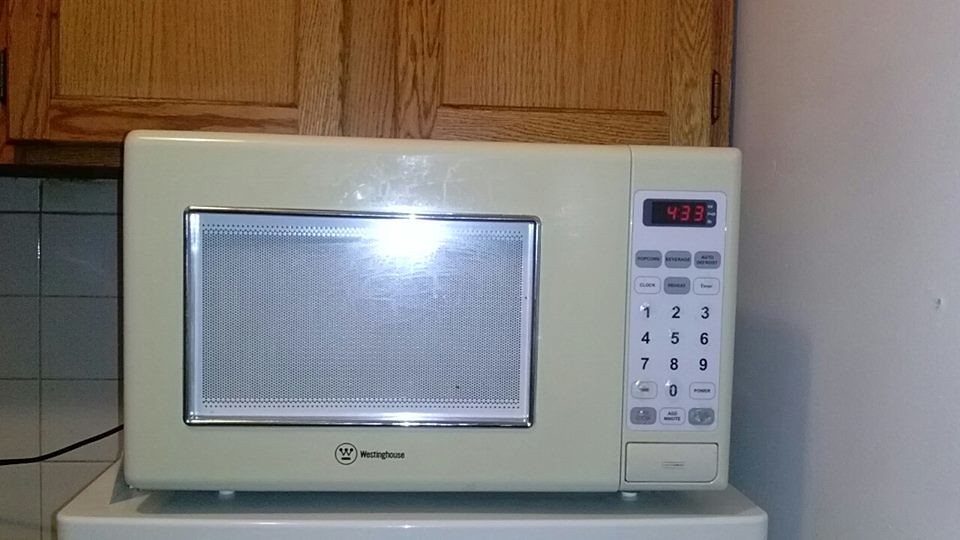The photograph depicts a close-up of a white Westinghouse microwave situated in a kitchen. The microwave, reflecting a bright light, prominently features a black and red digital clock displaying 4:33 at the top right of its control panel. Below the clock, a numeric keypad labeled 0 through 9 is visible, along with several other buttons that include a variety of white and gray tones. The appliance’s door, centered with a chrome-outlined window, occupies the left part of the microwave and has the Westinghouse logo and brand name situated below. 

The microwave sits atop a white, plastic-looking surface, which appears to be part of a kitchen appliance such as a fridge. A black cord trails off from the microwave's back toward the left, disappearing from view. The kitchen background includes a white subway tile backsplash with darker grout and wooden cabinetry consisting of a double cabinet hanging above the microwave. The right side of the microwave is adjacent to a white wall.